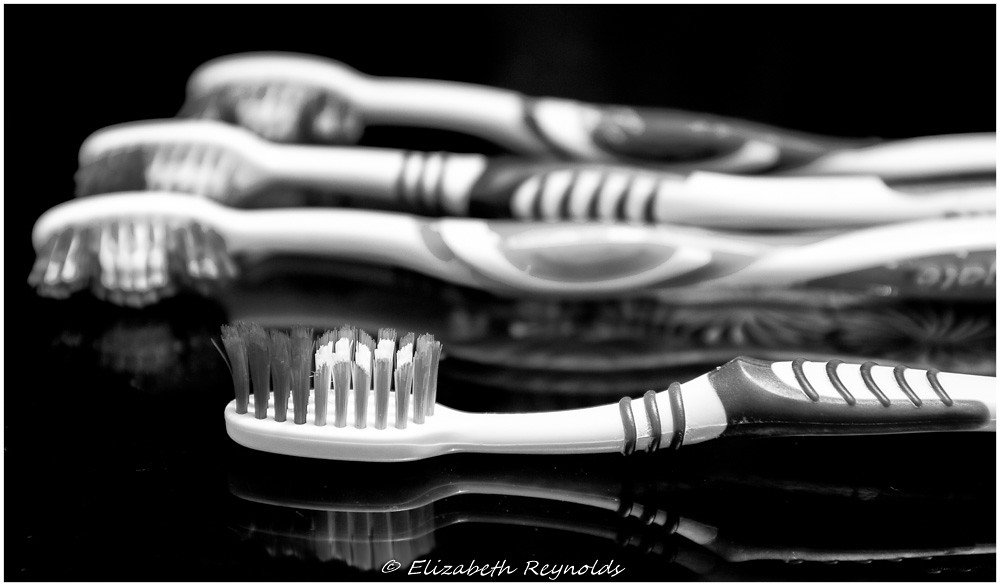In this black-and-white photograph, the focal point is a standard toothbrush laying on its back with its bristles pointing upwards. The toothbrush has distinctive dark gray bristles on top, lighter gray bristles on the sides, and white bristles in the center. Its neck features three lines for grip, along with additional lines down its center, and its handle is partially out of the right frame. The brush has rubber accents both on the top and the sides. Background toothbrushes, slightly blurred, form a group of three: one lays on its side with bristles facing towards the camera, while the other two, also on their sides, share this orientation. All toothbrushes rest on a highly reflective black marble countertop, creating clear reflections. A thin white border frames the photograph, and at the bottom center, the text "Copyright Elizabeth Reynolds" is elegantly inscribed.